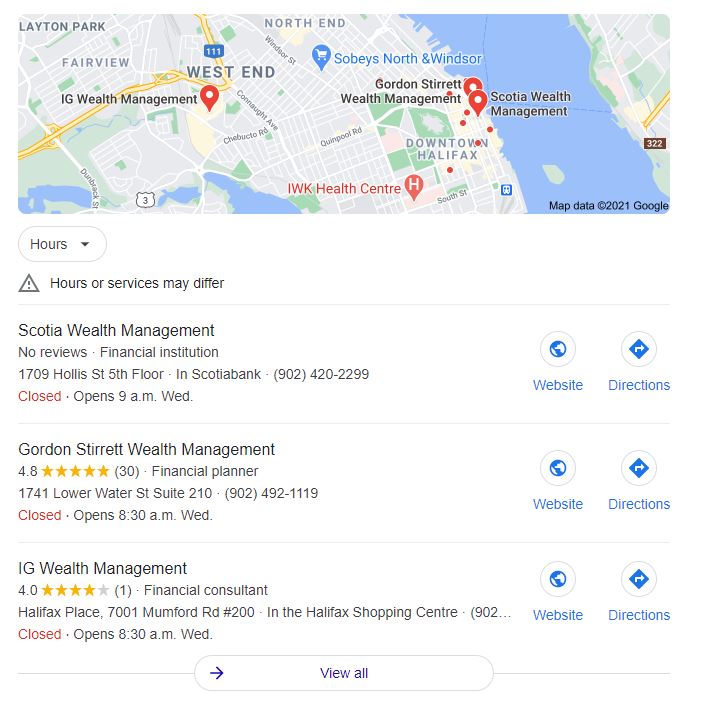At the top of the page, the image displays a detailed map of downtown Halifax, prominently featuring areas marked as West End, Fairview, North End, and IWK Health Center. The map is adorned with several pins, with red pins indicating specific locations such as IG Wealth Management and Scotia Wealth Management. A solitary blue pin identifies another place of interest. 

To the lower left corner of the map, a note reads "Map Data © 2021 Google," along with a disclaimer stating "Hours or services may vary."

Underneath the map, three search results for wealth management companies are listed:

1. **Scotia Wealth Management**
   - *Category*: Financial Institution
   - *Reviews*: No Reviews
   - *Address and Phone Number*: [Not specified in the prompt]
   - *Status*: Closed. Opens 9 a.m. Wednesday.
   - *Icons*: A globe icon labeled "Website" and a four-sided figure with an arrow pointing right labeled "Directions."
   
2. **Gordon Stewart Wealth Management**
   - *Category*: Financial Planner
   - *Rating*: 4.8 stars
   - *Address and Phone Number*: [Not specified in the prompt]
   - *Status*: Closed. Opens 8:30 a.m. Wednesday.

3. **IG Wealth Management**
   - *Category*: Financial Consultant
   - *Rating*: 4.0 stars
   - *Address and Phone Number*: [Not specified in the prompt]
   - *Status*: Closed. Opens 8:30 a.m. Wednesday.